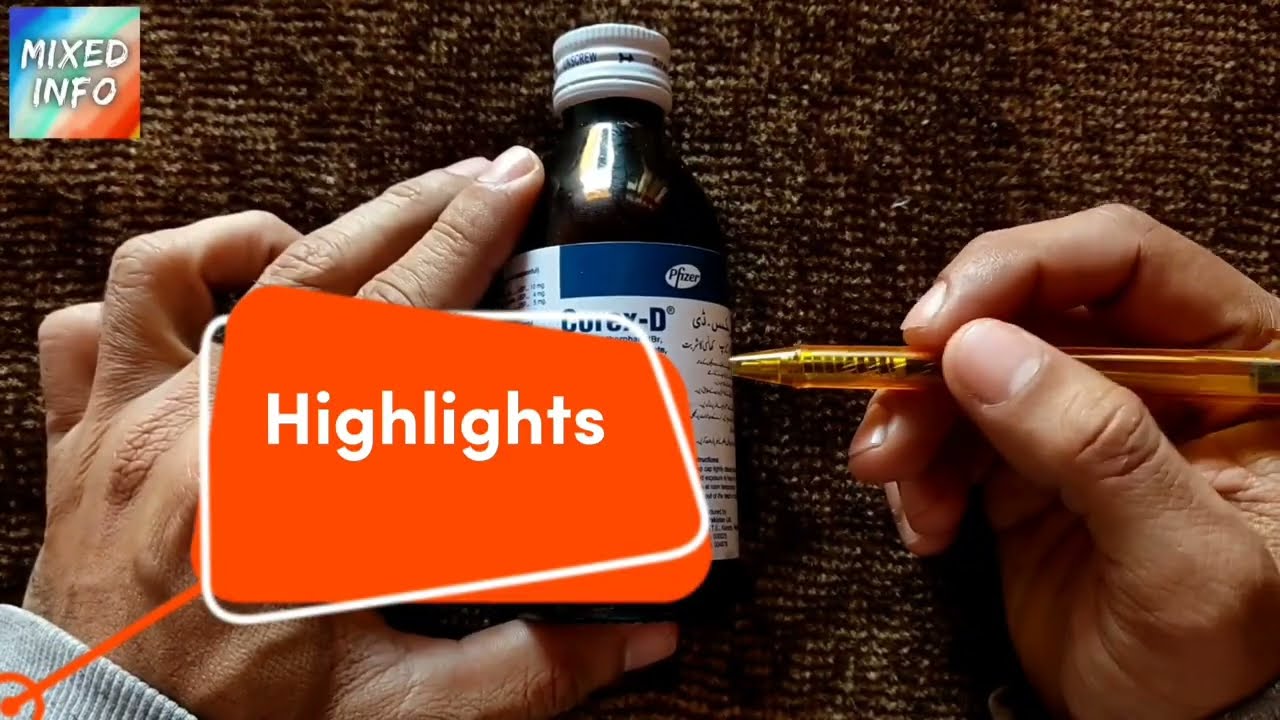In the image, two white hands are delicately holding a bottle of Pfizer medicine, identified by its characteristic blue stripe and white label, with the left hand gripping the bottle and the right hand writing on it with a yellow pen. The overall background is a brown and white patterned surface, possibly mimicking a work area. On the top left corner of the image, a square logo with a rainbow-colored background displays the text "Mixed Info" in white, capital letters. Centrally, there's a prominent orange rectangular banner with a white outline and the word "Highlights" written in white, commanding attention. The intricate visual composition reflects a blend of medical, informative, and possibly casual or hobbyist elements.